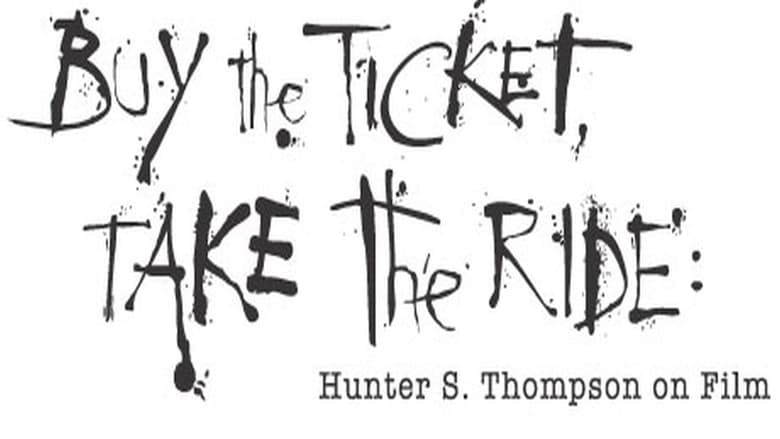In the center of a stark white background, the image features the text "buy the ticket," followed by a comma, and "take the ride," with a colon. These prominent lines are rendered in a creepy, hand-painted black font, with varying sizes of dots and splotches lending an edgy, unsettling vibe reminiscent of ink drips. Below this, in a regular typewriter-style font, the phrase "Hunter S. Thompson on film" is inscribed, also in black letters. The overall composition evokes a sense of eerie anticipation and pays homage to the iconic American journalist and author.